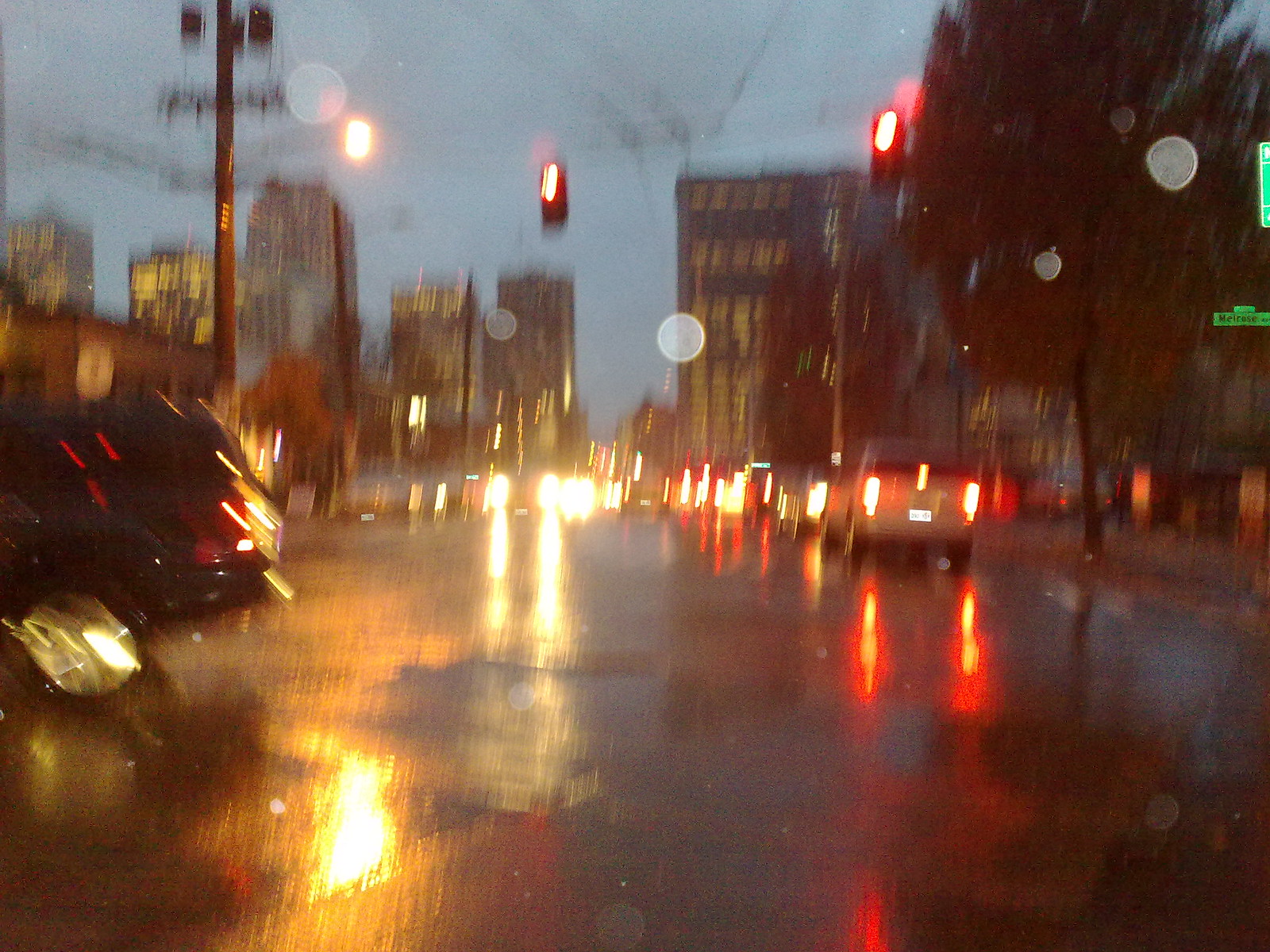This image depicts a blurred, rainy evening scene in a bustling American city with wet streets reflecting the various lights. In the foreground, several cars, including a noticeable pickup truck on the right, are stopped at a red light, their brake lights glowing vividly. Other vehicles' headlights beam from the opposite direction, accentuating the reflective wet ground. Overhead, traffic lights, and street lights dangle suspended on wires, casting a faint golden glow from some distant buildings. The image also features soaked sidewalks, a street sign for Melrose Ave in green, and a large tree to the right, partly obscuring a building. High-rise skyscrapers loom faintly in the distance against the evening's gray sky, contributing to the cityscape's overall ambiance. Despite the blur and water spots on the lens, the scene's details, from telephone poles and electrical wires to the orderly lined-up cars and the visible business fronts, paint a lively urban atmosphere.